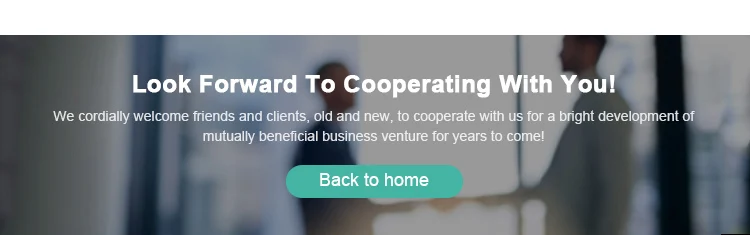In the background of this image, there's a banner with a gray, somewhat blurry appearance, signifying an office-like setting. At the center of the banner, two people face each other; the individual on the left stands against a slightly bluish tint, while the person on the right, who appears slightly taller, is positioned beside what looks like glass windows showing buildings outside. The pair seem to be engaged in a handshake, symbolizing cooperation. Overlaid on the image in white font is the text, "Look forward to cooperating with you. We will cordially welcome friends and clients, old and new, to cooperate with us for a bright development of mutually beneficial business ventures for years to come." Below this, a "Back to Home" button is centrally placed.